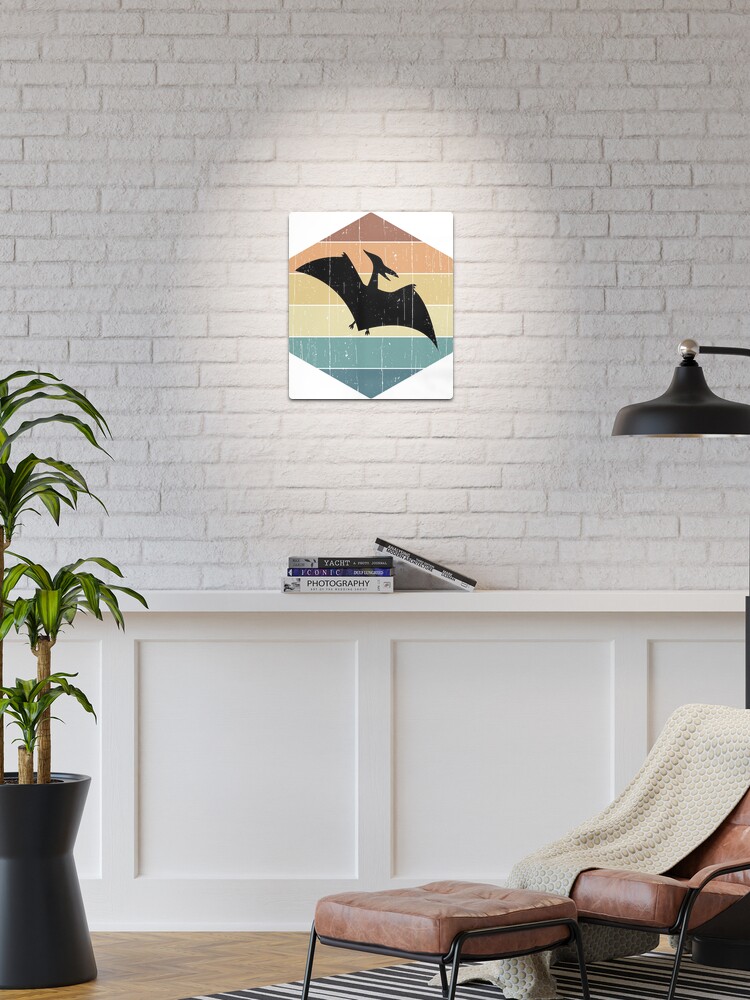The photograph depicts the interior of what appears to be a residential living space, boasting a striking white painted brick wall. Centered prominently on this wall is an eye-catching painting with a dominant diamond pattern. The diamond is composed of vibrant color bands that transition from the top-down: red, orange, yellow, pale yellow, teal, and aqua. At the heart of this geometric design is the black silhouette of a pterodactyl, its distinctive sharp beak and leather-like wings spread wide. Beneath this artwork, a white banister or shelf runs horizontally, adorned with several books. To the left of the banister stands a potted plant, adding a touch of greenery to the setting. On the right, a small brown leather chair with a matching footstool rests atop a black-and-white striped rug, with a cozy blanket draped over them. A hanging black lamp looms above the seating area, contributing to the room's inviting ambiance. The floor appears to be wooden, adding warmth to the overall aesthetic.